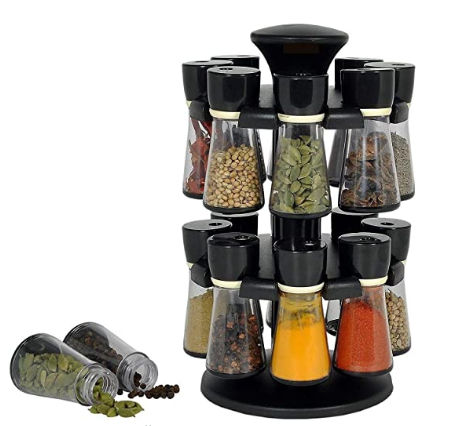This image showcases a circular, two-tiered spice rack set against a plain white background, likely intended for a product highlight. The rack, positioned on the right side of the image, holds multiple clear glass jars filled with various spices, seeds, and powders in colors such as green, black, brown, yellow, orange, and red. Each jar features a black lid, which may function as either a shaker or grinder. The design allows the rack to spin around a central rod, providing easy access to the different spices. On the bottom left, two of these glass jars are seen tipped over, with their contents spilling out, illustrating ease of use and accessibility. The clean, text-free background and arrangement suggest a setting that could be either a kitchen or a stock image for commercial purposes.